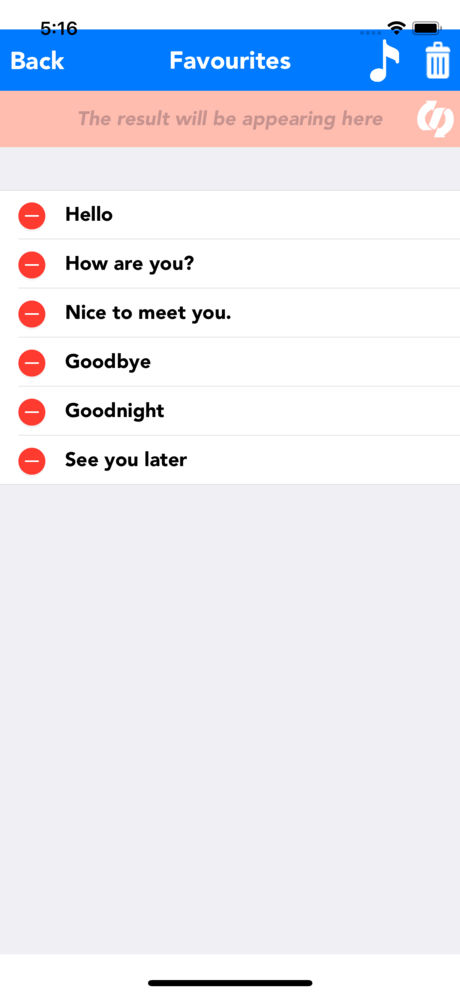This is a detailed vertical smartphone screenshot. The image appears to be taken against a computer screen backdrop, primarily white, with a mix of other background elements. 

At the top, a thick blue rectangular bar stretches across the screen. Positioned at the very top, partially overlaying the blue onto the white of the computer background, the time reads "5:16" in black. Adjacent to the time, there is a Wi-Fi icon followed by a battery life icon, both similarly straddling the blue and white portions. 

In the blue bar, to the left, the label “Back” is written in white, while the center displays the word "Favorites." On the right-hand side, there are two icons: a music note and a trash can. 

Below this, a salmon-colored rectangular highlight states, "The result will be appearing here," accompanied by two white twisty arrow icons on the right. Subsequently, a smaller gray strip spans the screen before transitioning to a section featuring numerous white strips, each separated by thin gray lines. Every strip contains a red circle with a white horizontal line through it, indicating an action yet to be specified.

The first strip reads, in black text, "Hello," followed by sequential strips with the phrases: "How are you," "Nice to meet you," "Goodbye," "Goodnight," and "See you later." 

At the very bottom, there is a plain gray box without any text, bordered underneath by a black line that crosses just below the middle of this gray square. This composition suggests a user interface, possibly from an application or a settings menu, showcasing selectable options or commands.